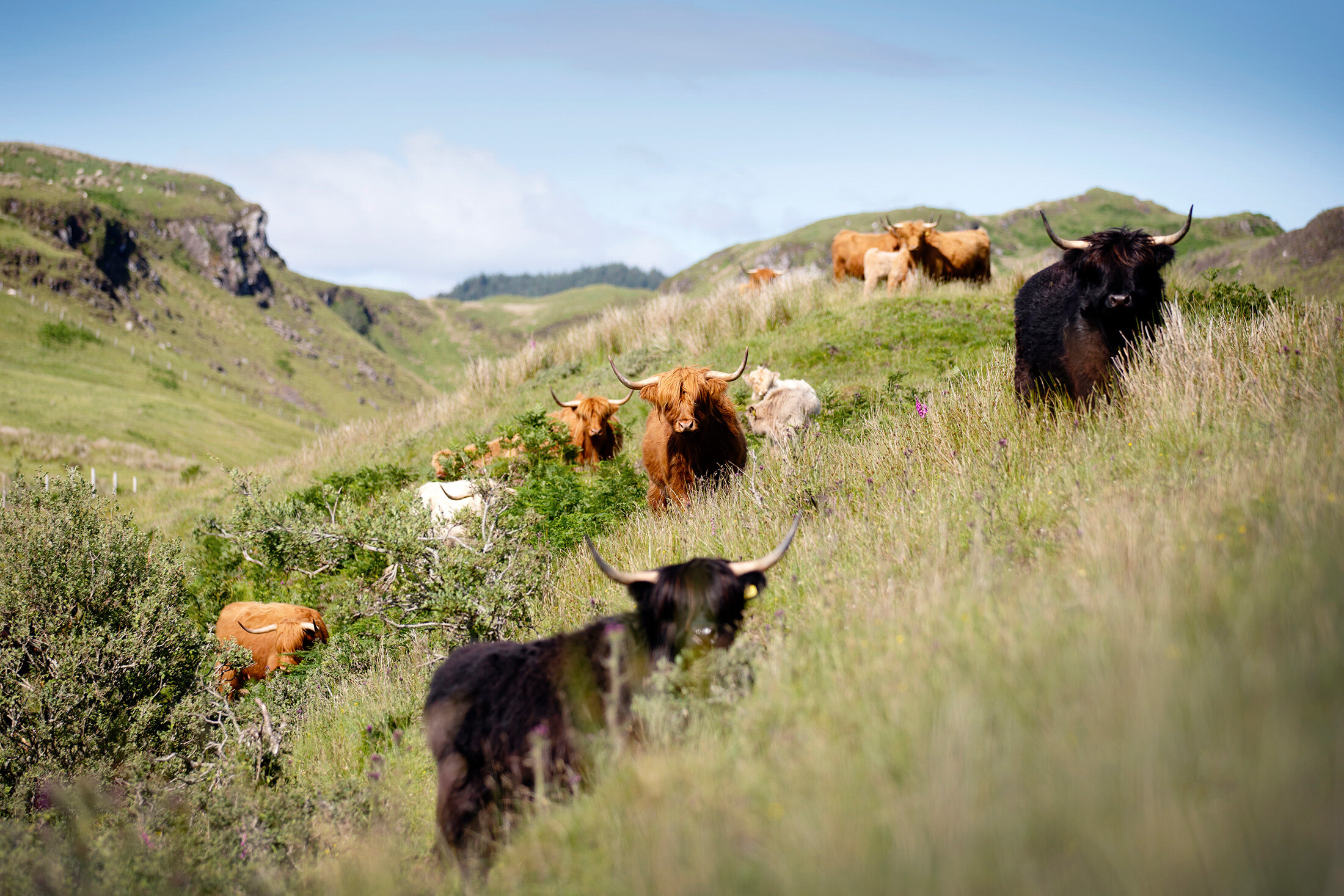The image captures a serene, large field with very tall, green grass, nearly reaching up to the shoulders of the animals roaming through it. In this photograph, a number of oxen with large horns and a mix of black and brown fur are grazing and resting in the lush grass. Notably, two black oxen with imposing horns stand closest to the camera, gazing directly towards it. Further in the background, centered in the image, a larger brown ox is prominently visible, with another smaller brown ox slightly to its left. Among them, there appears to be some white-furred animals, possibly smaller calves or sheep, enhancing the pastoral vibe of the scene.

Off to the left, large bushes add texture to the landscape, while further back, rocky hills rise up, hinting at a more rugged terrain. Beyond these hills, the backdrop transitions into a dense forest that stretches out under a blue sky scattered with white clouds. The high-quality lens used for this photograph focuses crisply on the central area, providing sharp details of the oxen, while the foreground and background subtly blur, emphasizing the depth and tranquility of this rustic setting.